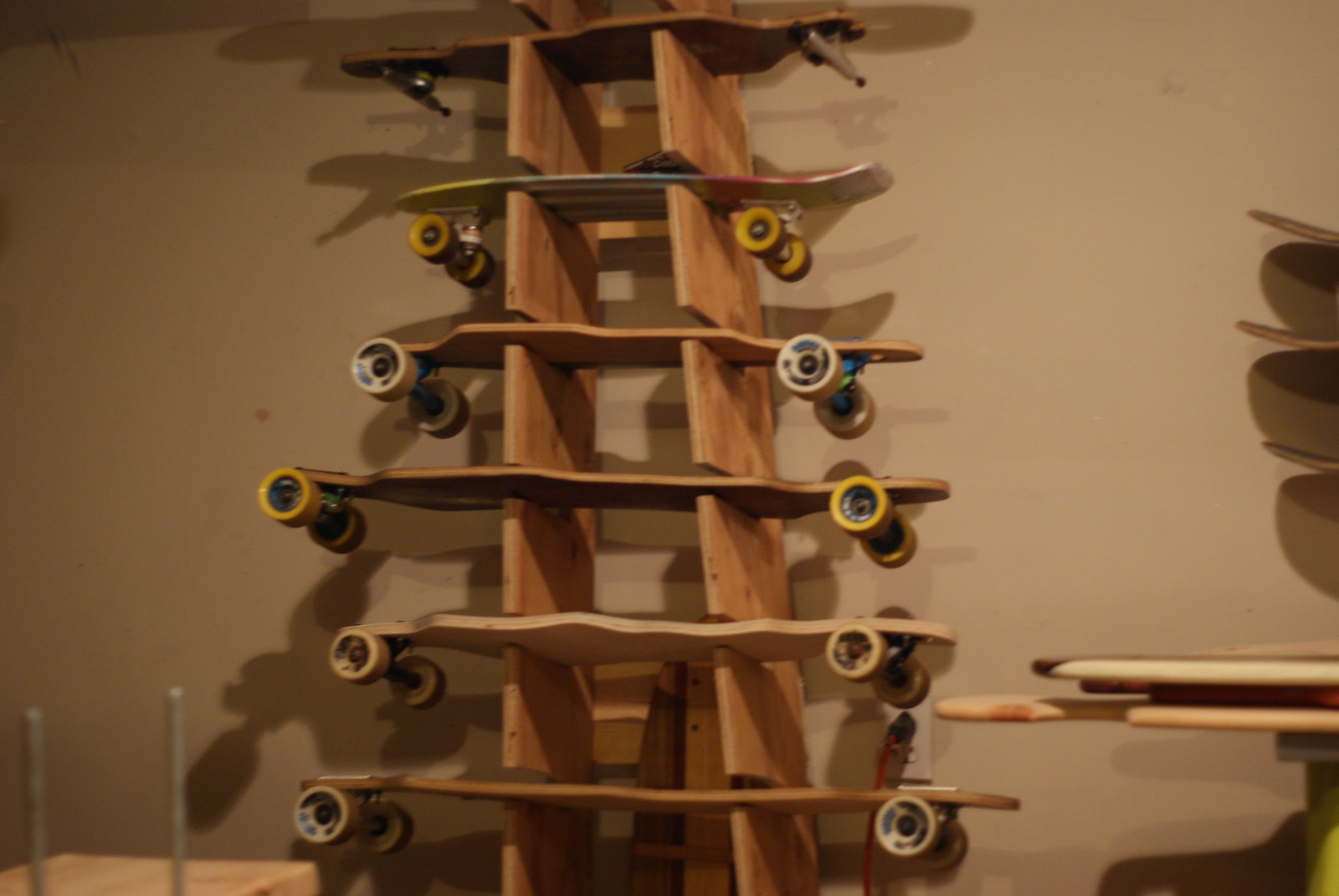This image showcases a wooden rack structured to hold six skateboards of varying sizes, all arranged within precisely cut divots or slits. The skateboards are placed from longest at the bottom to smallest at the top, resembling a tower. The top skateboard has tracks but no wheels, while the second from the top, a small penny board, is multicolored with wheels. Moving downward, the third skateboard is a regular longboard with white wheels, and below it, a significantly longer skateboard with yellow wheels. The fifth skateboard is slightly shorter, also with white wheels, followed by another equally long skateboard at the bottom, featuring similarly colored white wheels. The scene is set against a tan-beige wall, with the light casting distinct shadows of the skateboards onto the wall. To the right, partial views of surfboards are visible, stored in a similar type of holder. Glimpses of metal dowels can be seen towards the lower right corner, adding to the image's detailed composition.